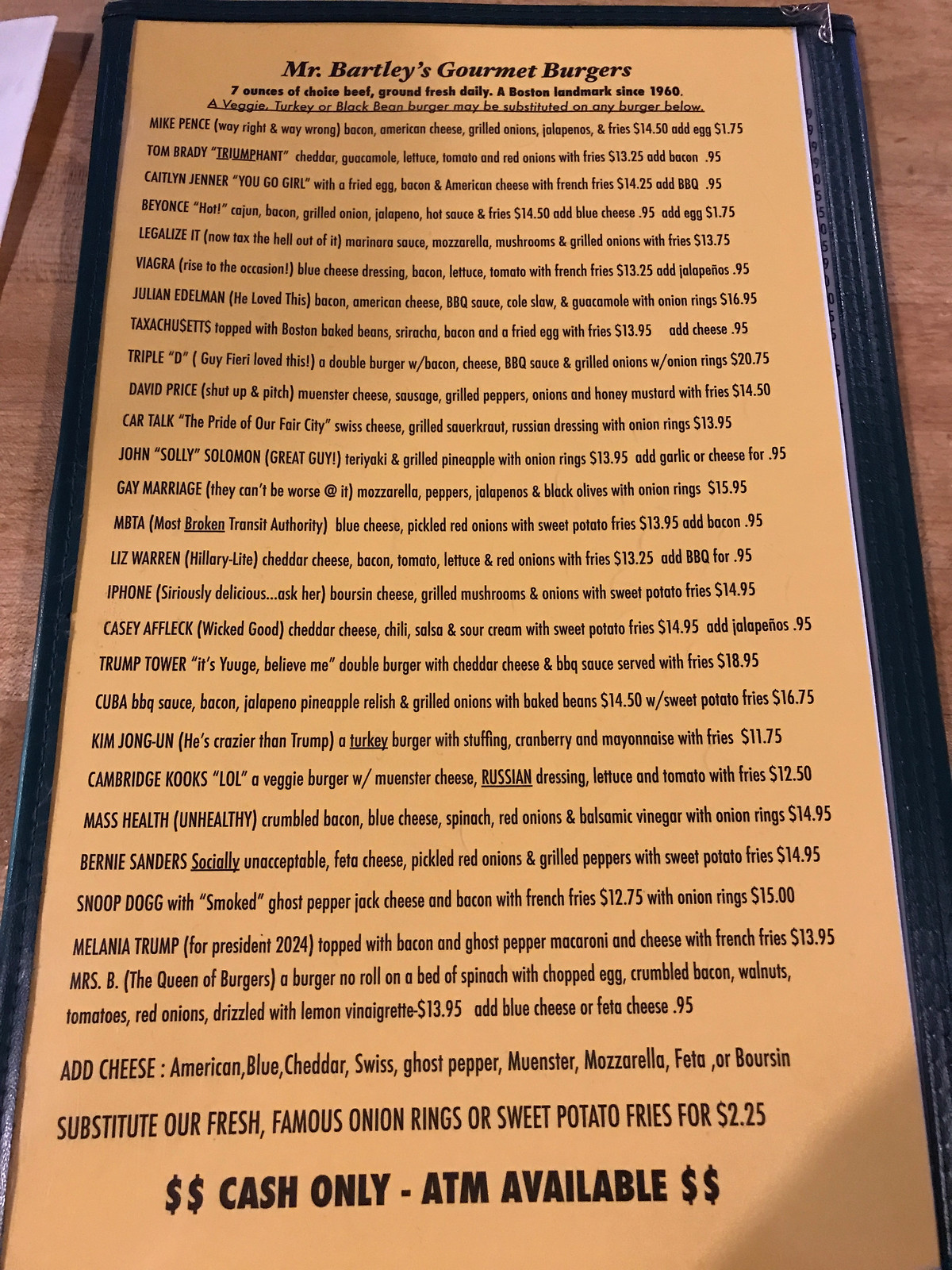The image depicts a detailed menu resting on a basic wooden table, which features a napkin in the background. The menu, encased in plastic, showcases a peach-colored background with black lettering that reads "Mr. Bartley's Gourmet Burgers." Although the angle of the photo makes the text challenging to read, the menu lists an eclectic range of burger names inspired by notable personalities and themes. These include "Mike Pence," "Caitlyn Jenner," "Beyoncé," and more intriguingly named options such as "Legalize It," "Viagra," "Julian Elderman," "Taxa Shoe Sits," "Triple O," "David Pike," "Car Talk," "John Solomon," "Gay Marriage," "Metta," "Trump Tower," "Casey Affleck," "iPhone," "Liz Warren," "Cuba," "Kim Jong Un," "Cambridge Kooks," "Mass Health," "Bernie Sanders," "Snoop Dogg," "Melania Trump," and "Mrs. B." The diverse and creative names suggest a playful and humorous take on the gourmet burger offerings at Mr. Bartley’s.